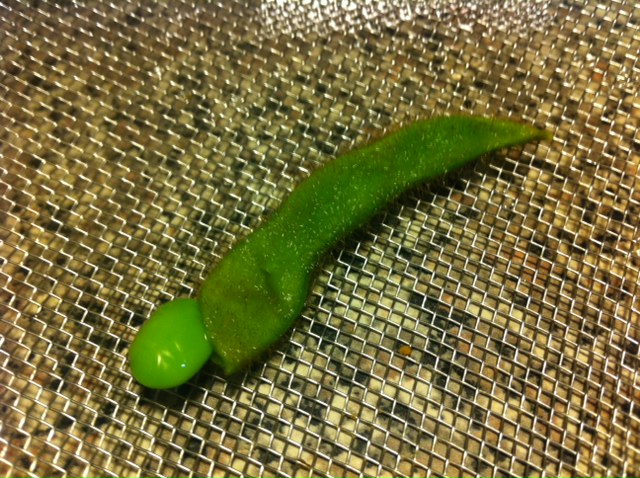In this highly detailed and close-up photograph, a single green pea pod is prominently displayed, set against a beige-brown backdrop. The surface atop which it rests appears to be a fine wire mesh or grid, potentially metallic and positioned diagonally across the image. This grid imparts a diamond pattern when viewed through the semi-translucent pod, adding to the intricate texture of the scene. The pea pod itself curves gracefully from the bottom left towards the top right, resembling the beak of a bird. Detailed textures are visible on the pod, including its shiny, washed surface and fine, hair-like structures. A single pea, glossy and vibrant, peeks out from the opened end of the pod on the left-hand side, almost completely detached yet still clinging delicately to its shell. The careful composition and meticulous focus make the individual details — from the sheen of the pea to the wire grid beneath — distinct and visually striking.